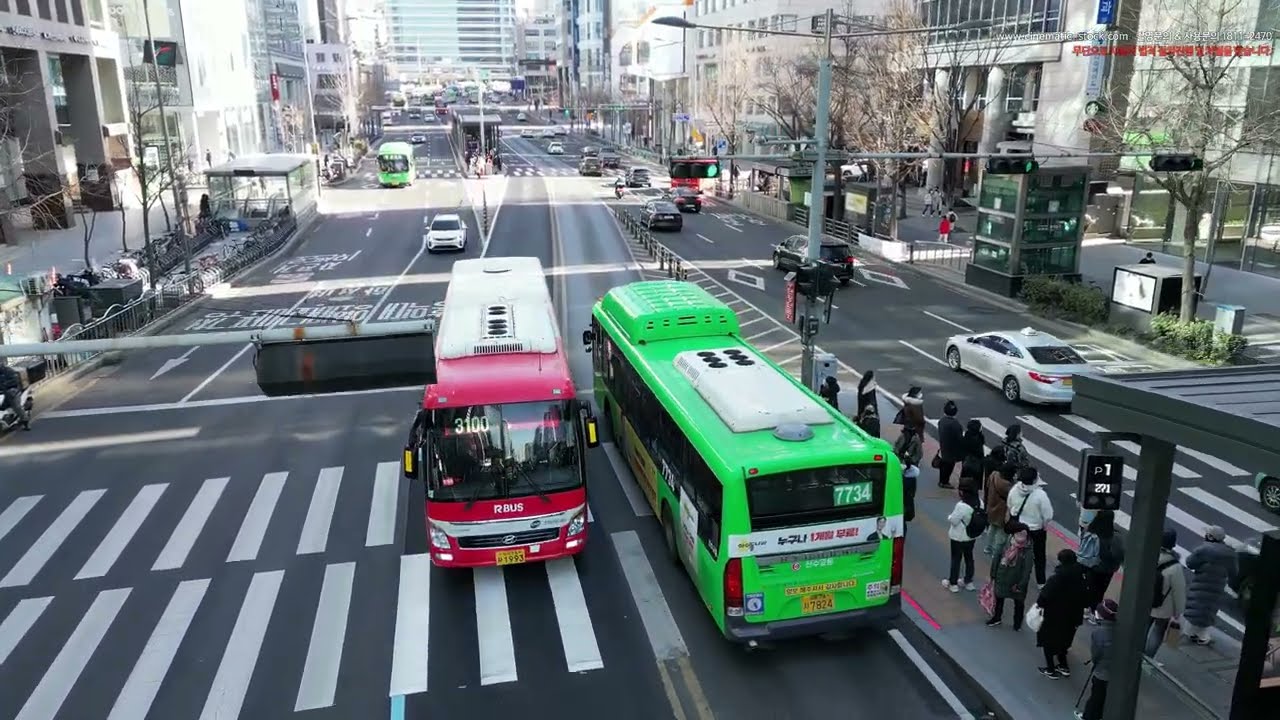The image captures an aerial view of a bustling urban cityscape centered around a busy intersection. The downtown scene is framed by tall glass buildings, with seven lanes of traffic flowing through—three lanes heading north and four heading south. At the focal point, two buses are passing each other; a large green bus with a white top marked with the number 7734 is heading upward, while a red bus with a similar white top is moving downward. Both buses traverse a crosswalk, with a group of people standing on a central island, seemingly waiting for buses heading in either direction. The pavements are populated with pedestrians and various cars, adding to the dynamic city life. The image is vibrant with colors including green, white, red, black, gray, yellow, blue, pink, purple, and light blue. Small text, possibly Japanese, is present but unreadable, contributing to the urban ambiance.